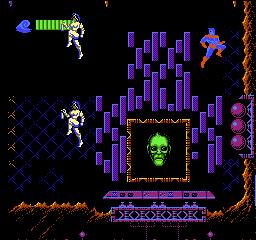In this screenshot from an 8-bit video game, the focal point is a green face prominently displayed in a square frame at the center of the screen. This face is enclosed by a squiggly, rectangular border. Surrounding the central figure are purple rectangles positioned on the left, right, and top sides, with a purple base situated underneath the rectangle.

To the left of the central face, a white figure wearing a blue helmet is captured mid-jump in the air. This figure stands out against a black background speckled with blue X-shaped patterns, as well as some lighter X's off to the left. Directly above this jumping figure, another similar character is depicted in an identical jumping pose.

On the right side of the image, a figure with blue clothing and darker skin tone faces a different direction, adding varied movement to the scene. The outer edges of the screen are tinted with a brown, rocky texture.

Adjacent to the right wall, three distinct purple orbs are attached, contributing to the level's intricate design. In the upper right corner, an indicator comprised of several vertical green rectangles extends to the right. To the left of these rectangles, a bluish "whoosh" effect adds dynamic energy to the display. The overall background remains mostly black, with intermittent blue X textures breaking up the darkness.